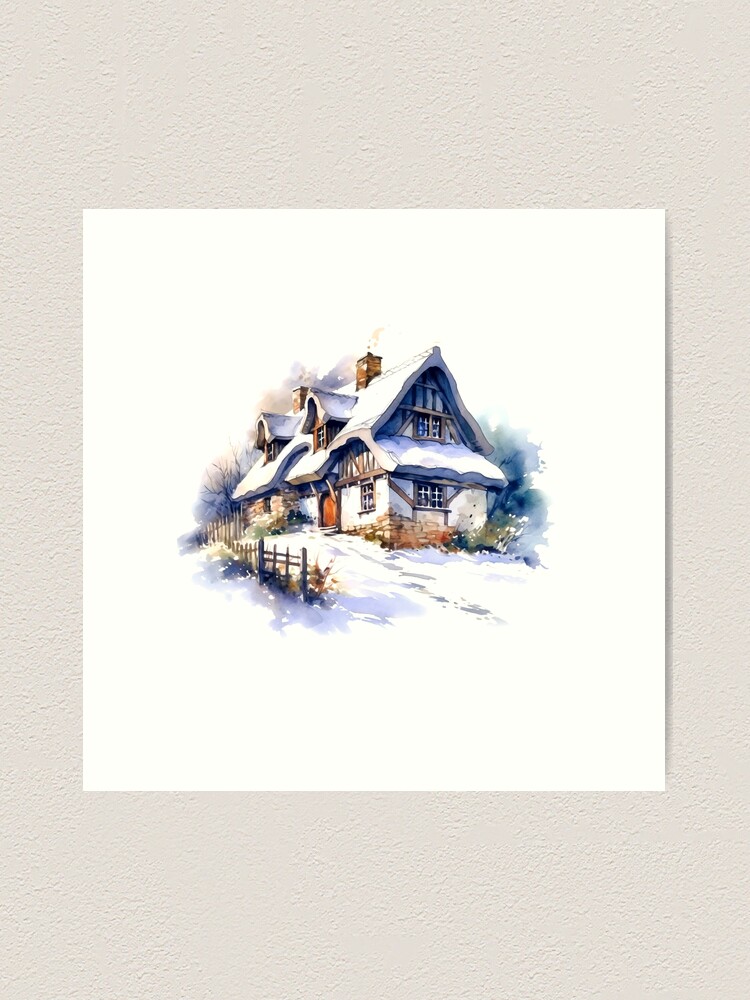This detailed painting depicts a cozy two-story house perched atop a steep, snow-covered hill, giving it a picturesque wintery charm. The house, adorned with a golden-brown or red front door, exudes warmth with smoke billowing from its brick chimney. Snow blankets the entire rooftop, and the exterior of the house features shades of blue, purple, and orange paint that subtly bleed onto the sides of the painting, adding a unique artistic touch. A well-trodden path with visible footprints leads up the hill to the front steps, passing through a wooden picket fence. On either side of the house, leafless trees stand stark against the white landscape, while a small garden or bushes nestle up beside the building. The windows are framed with wooden beams, further enhancing this serene winter scene.